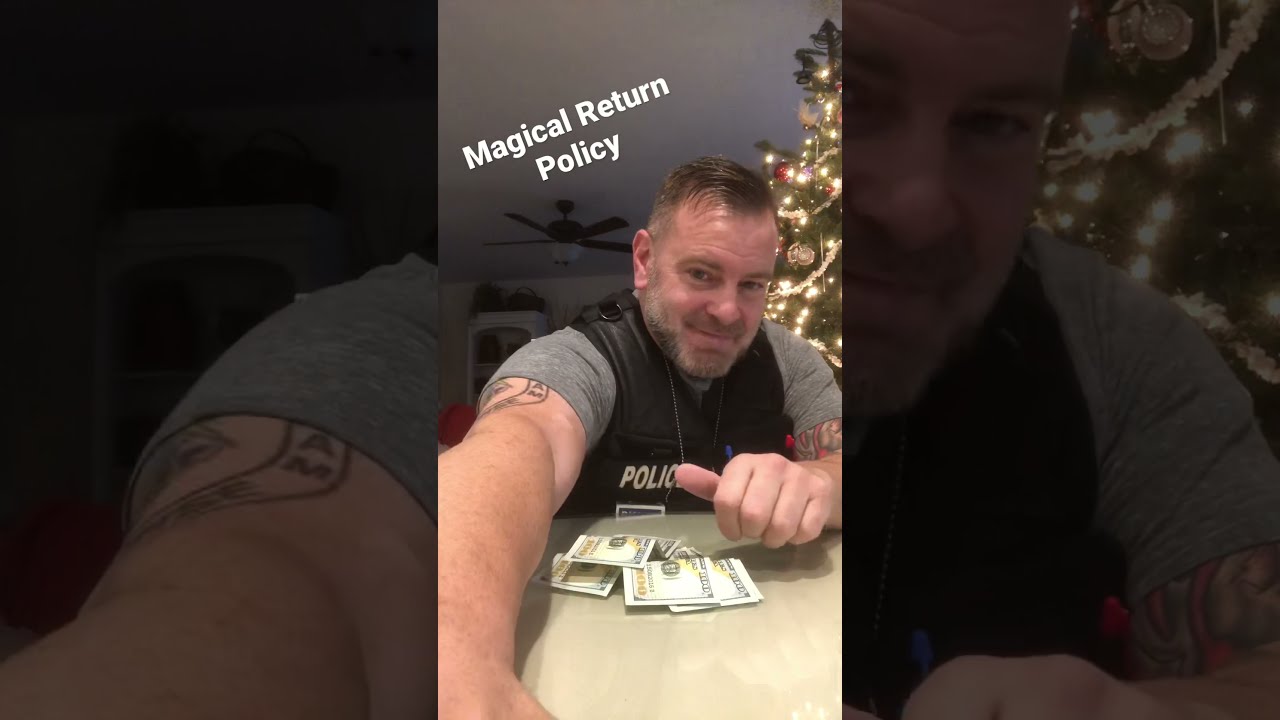The image is a composite photograph presented in a horizontal rectangular format, divided into three sections (left, middle, and right). The main focus is a central vertical cell phone-style picture of a middle-aged white man, overlaid on a faded, zoomed-out version of the same image that fills the background.

In the central section, the man, who has stubble on his face, is seated at a table and facing the camera. He is wearing a black vest resembling a police or bulletproof vest with the word "POLICE" written on the right chest area, over a short-sleeved gray shirt. His right arm extends forward, partially out of the frame, revealing a tattoo on his upper arm that peeks out from under his sleeve. His left hand rests on the table in front of him, near a stack of hundred-dollar bills. Above him, on the top left, the phrase "magical return policy" is written in white text. 

The background visible behind him includes a variety of household items that provide context to the scene: a lit Christmas tree over his left shoulder, a ceiling fan over his right shoulder, and a bookshelf along the wall, suggesting a home setting.

The left and right sections of the image depict darker, slightly different angles of the same man. On the left side, the focus is on his tattooed right arm and the sleeve of his gray shirt. A white hutch with various items adds subtle detail to the background. The right section shows a partial profile of his face with the Christmas tree again visible over his left shoulder and his left hand's knuckles cropped at the bottom of the image.

Overall, the photograph captures the man in a dimly lit home environment, highlighting specific elements like his tattoo, police vest, stubble, and the festive background details.